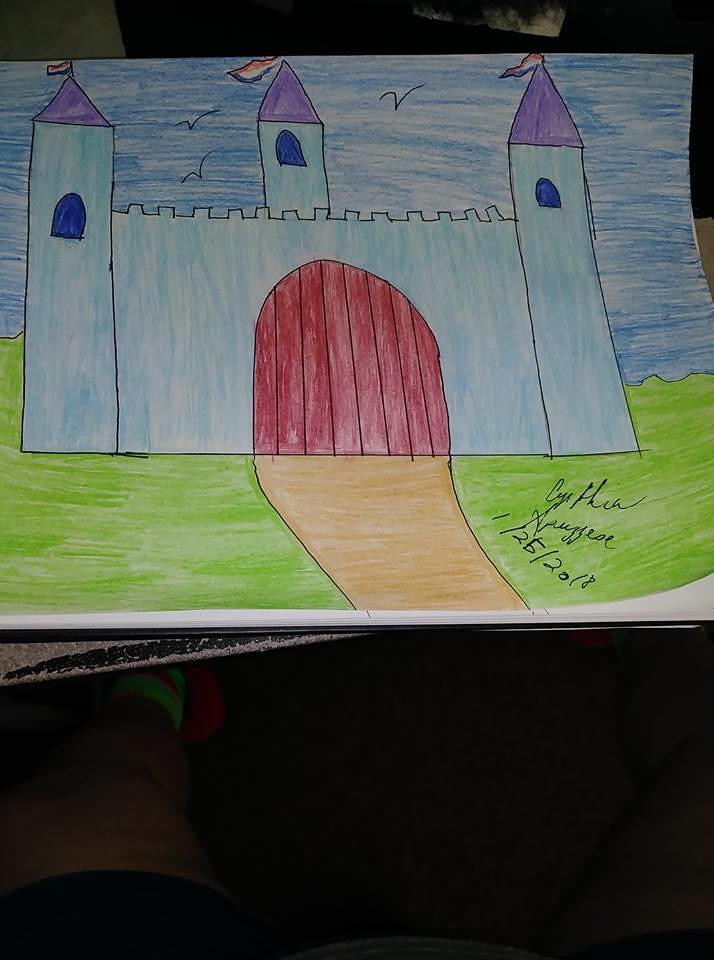A meticulously colored drawing showcases a majestic castle, rendered with vivid Crayola hues. The fortress features a square front façade, anchored by two imposing towers at each corner. In the background, another tower rises above the structure, creating a sense of depth. Each of the triangular tower roofs is adorned in a vibrant purple, crowned with fluttering flags. The castle entrance boasts a bold red door, and a brown pathway leads from it, slicing through the lush, green landscape surrounding the castle. The artist has signed the piece and dated it from 2018, adding a personal touch to this charming illustration.